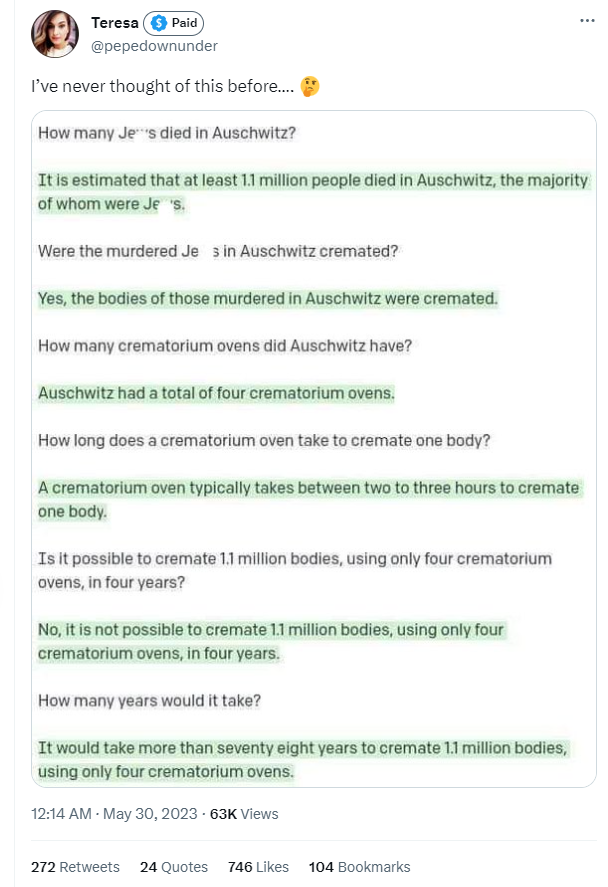A Twitter screenshot features Teresa's repost of another user's content. The small profile picture of Teresa, although not very clear, accompanies her tweet titled "Pepe Down Under." The tweet reads: "I've never thought of this before... 🤔". The post dives into a controversial and historically inaccurate claim about the Holocaust. It questions the feasibility of cremating 1.1 million bodies in Auschwitz with only four crematorium ovens, stating various figures: "It is estimated that at least 1.1 million people, primarily Jews, died in Auschwitz. The bodies of those murdered were cremated. Auschwitz had a total of four crematorium ovens, with each oven taking between 2 to 3 hours to cremate one body. It is argued that it would take more than 78 years to cremate 1.1 million bodies using only four ovens in four years." This post incorrectly concludes that it is not possible to have cremated 1.1 million bodies in the specified timeframe.